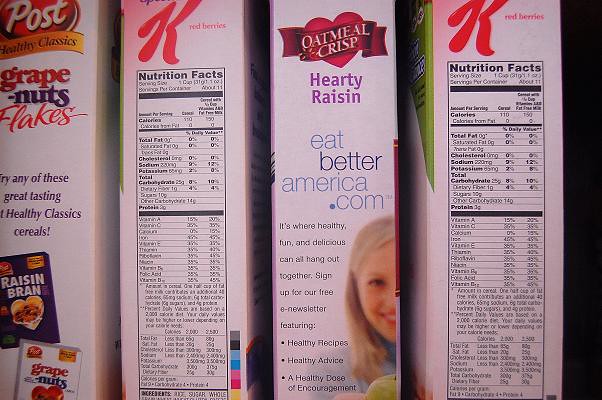The photograph features the sides of four distinct cereal boxes, each of different brands and types. From left to right, the first box is Post Grape Nuts Flakes, showcasing its advertising panel with claims of being great tasting and a healthy classic. The second and fourth boxes are Kellogg's Special K Red Berries, both displaying their nutritional information with tables of vitamins and fats. The third box is Oatmeal Crisp Hearty Raisin, also featuring an advertising panel that promotes healthiness, directs to eatbetteramerica.com, and includes a sign-up for a free e-newsletter full of healthy tips and recipes. This Oatmeal Crisp box has an image of a smiling woman with medium-length blonde hair, wearing a light blue sweater and holding a green apple. All the boxes share a predominantly white color scheme with red logos, and some display pictures of the cereal while others are focused on nutritional facts and ingredients.